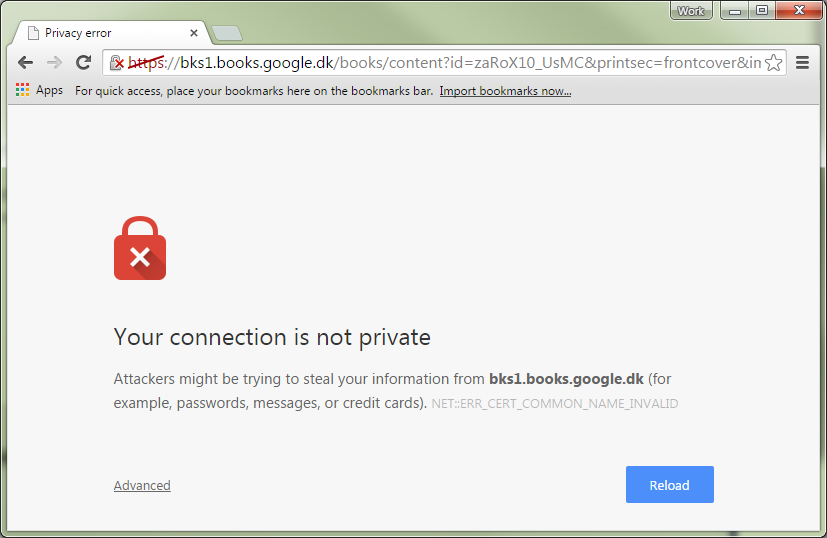This image depicts a web browser displaying a privacy error message, with several key elements highlighted. At the top, there's a bookmark bar containing a folder icon labeled "Privacy Error." The URL shown reads "bks1.books.google.dk" suggesting the page pertains to Google Books' content.

Below the bookmark bar, there is a colorful box labeled "Apps," with a message prompting users to place bookmarks on the bookmarks bar or to import bookmarks. However, due to the privacy error, a small, red, clutch purse-shaped icon with a white 'X' in its center appears, signaling that "Your connection is not private." The error message warns that attackers might be attempting to steal information such as passwords, messages, or credit card details from the site "bks1.books.google.dk."

The details of the certificate are partially visible, showing fields for "Common Name" and "Valid." At the bottom, there are two buttons: a blue "Reload" button to retry accessing the site, and an "Advanced" button on the far left to obtain more information about the error. 

In the top-right corner of the image, standard window control buttons are visible, including the close, minimize, enlarge, and close buttons again, facilitating standard browser window operations.